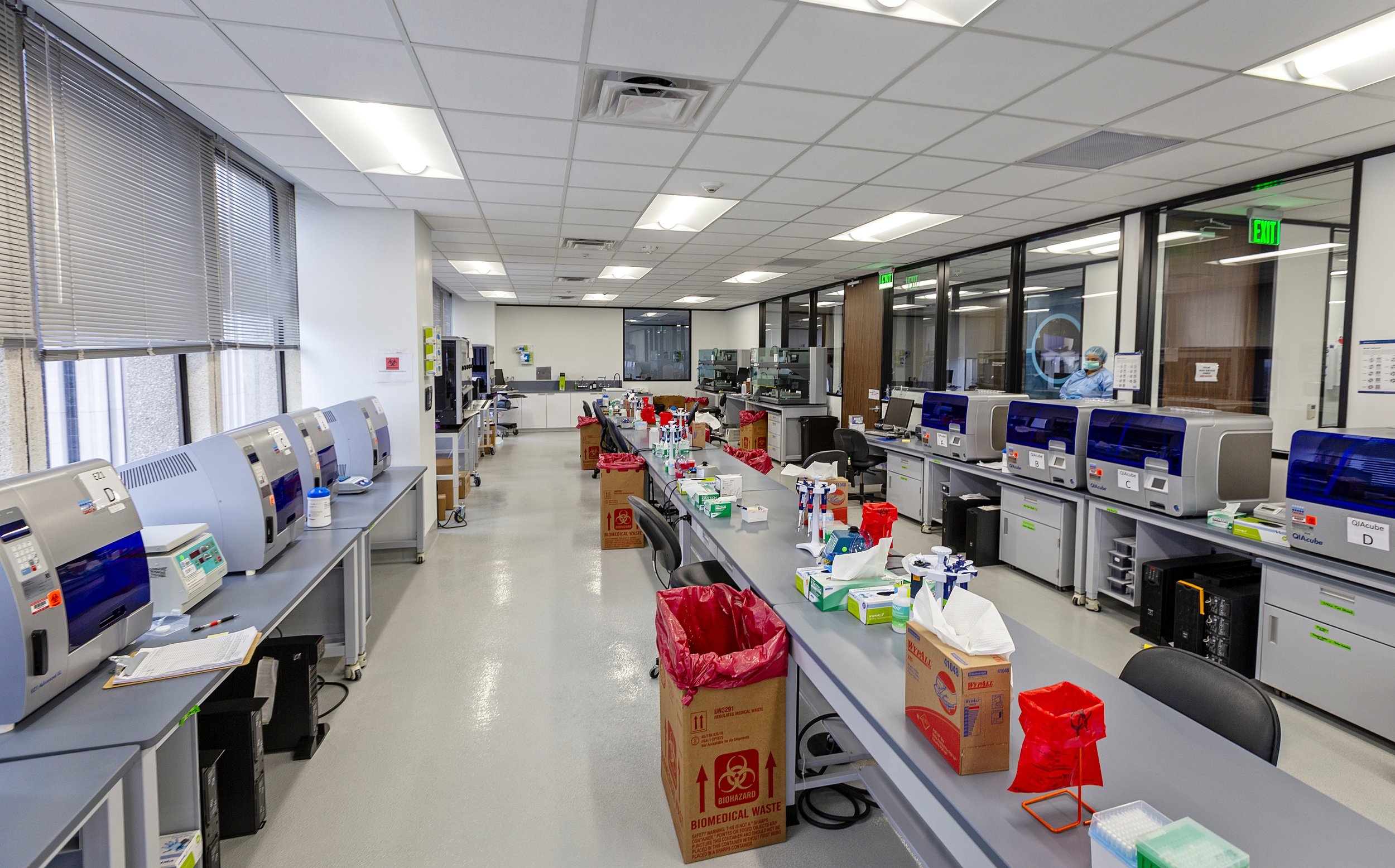The indoor photograph depicts a large medical laboratory with a sterile, organized environment. The lab features three expansive grey countertops—two along the walls on the left and right sides, and one running down the middle. All the countertops share a similar design, with light grey bases and darker grey tops. The countertops are populated with numerous large, rectangular laboratory devices, each featuring a distinctive blue panel of glass. Scattered across these surfaces are various pieces of lab equipment including boxes, drawers, gloves, and paper towels.

Biohazard containers are prominently displayed throughout the space, easily identifiable by their red bags and biohazard symbols. Additionally, there are smaller biohazard stands with red bags positioned on top of the counters. The walls and floor of the lab are both white, enhancing the sterile aesthetic.

On the left side, there are windows offering views to the outside, while windows on the right side look into an adjacent hallway. The ceiling is a standard drop ceiling with fluorescent lights, and there are visible exit signs in green. In the background, a person dressed in blue scrubs or a sterile gown, with a blue hair net and a mask, can be seen working, adding to the professional and clinical atmosphere of the laboratory.